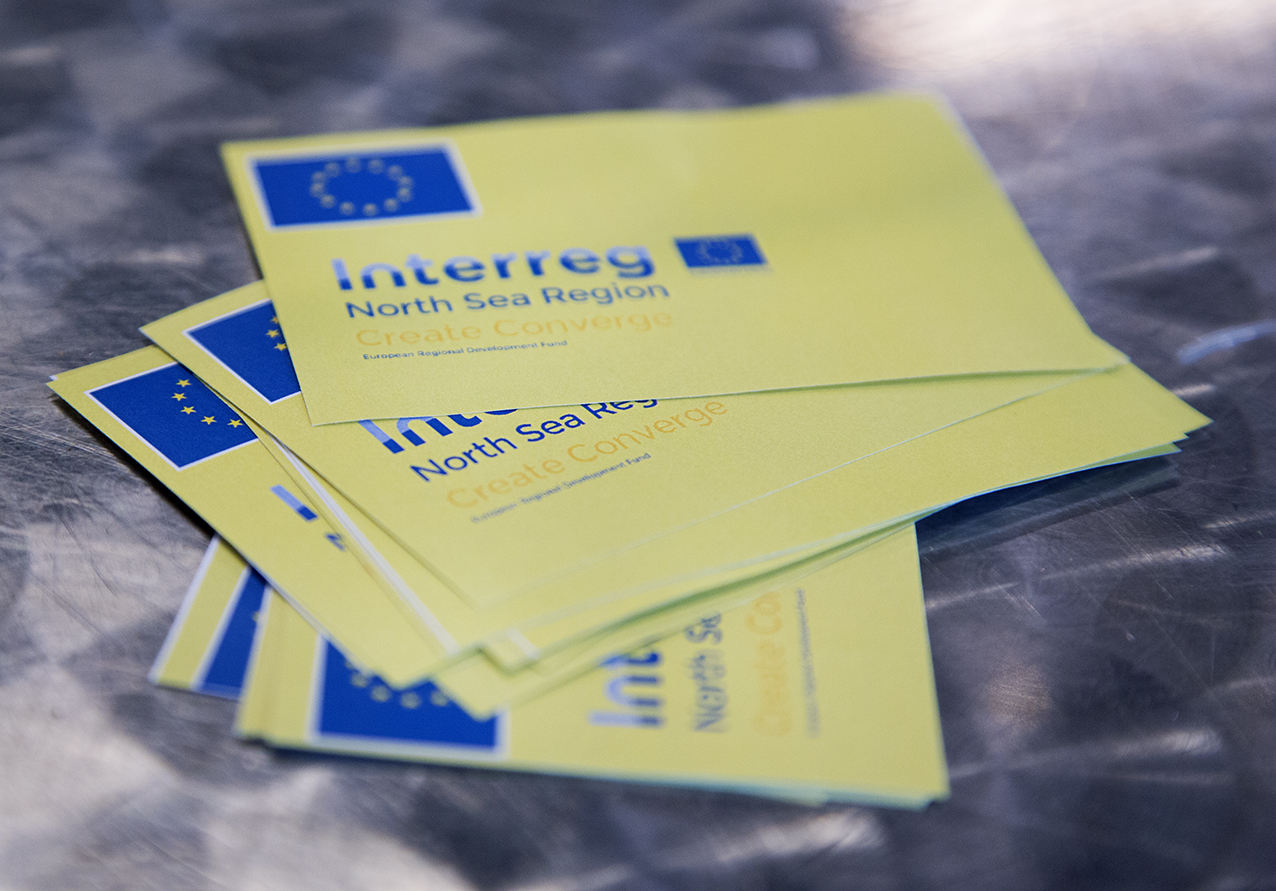The image depicts a neat stack of identical business cards displayed on a black, slightly speckled table. Each card is a vibrant yellow with a prominent blue box in the upper left-hand corner, featuring a circle of yellow dots within it. To the right of this blue box, there is an identical smaller blue box with yellow dots. The cards are slightly fanned out, revealing the printed details. The text "Interreg" appears in a gradient blue font, fading from darker at the top to lighter at the bottom, followed by "North Sea Region" in solid blue text. Below that, the words "Create and Converge" appear, written in yellow text. The stack appears to contain approximately 10 to 15 cards, all featuring these same elements and laid out orderly on the table.